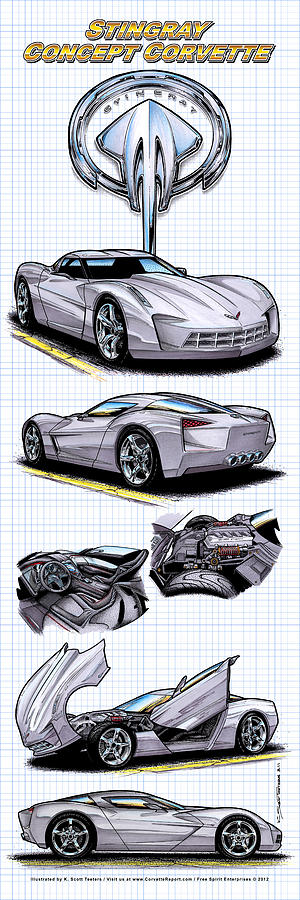This portrait-oriented computer-generated illustration showcases a Stingray Concept Corvette. The background features numerous blue horizontal and vertical stripes against a white backdrop. At the very top, in the center, there are two lines of text in yellow and red that read "Stingray Concept Corvette," followed by a silver emblem of a stingray logo. Below this, the image is divided into vertical segments, displaying various views of the car on a yellow base. 

The first vertical picture depicts the front view of a light pinkish-purple or silver-gray Corvette, noted for its distinctive chrome wheels and four exhaust pipes. The next image shows the rear view of the same car. Following these, there are two interior images displaying detailed depictions of the steering wheel and the instrument panel, indicative of the car's conceptual design. 

Further down, there are images showing the car from a side perspective with the hood open and the door lifted sideways, which gives a unique vertical opening mechanism. Finally, the bottom part of the illustration includes two profile views of the Corvette from different angles—the front left with the hood up and the door open, and another full side profile. Small black text is present beneath the final image, although it is difficult to read. The entire illustration has a hand-drawn aesthetic, though it appears to be created using computer-aided drafting software.